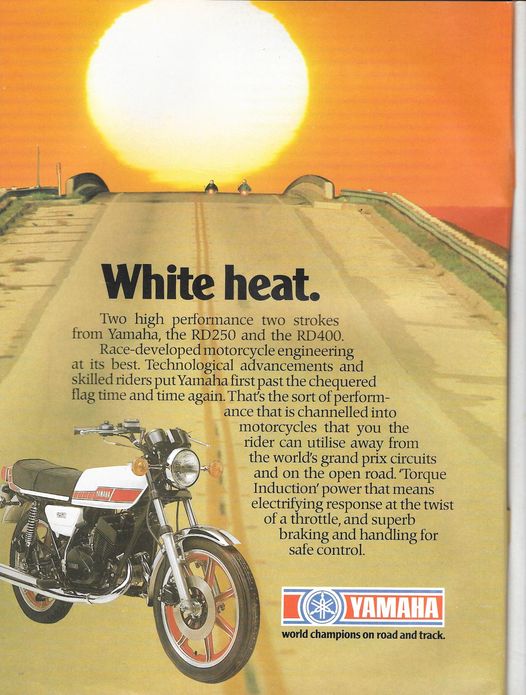This image is a detailed advertisement for Yamaha motorcycles, entitled "White Heat." The page-sized drawing features a motorcycle prominently positioned in the lower left corner, detailed in white with an orange stripe and a black seat. The bike is set on a bridge with a brown road that leads into the horizon. A large, intense yellow sun at the top is surrounded by vivid shades of orange and red, creating a striking sunset scene. On the horizon, two additional motorcycles ride into the distance. 

The text, centered in bold black letters, reads "White Heat" at the top, followed by "Two high-performance two-strokes from Yamaha, the RD250 and the RD400. Race-developed motorcycle engineering at its best, technological advancements, and skilled riders put Yamaha first past the checkered flag time and time again. That’s the sort of performance channeled into motorcycles that you, the rider, can utilize away from the world's Grand Prix circuits and on the open road. Torque Induction power means electrifying response at the twist of a throttle and superb braking and handling for safe control."

In the lower right corner, there's the Yamaha logo in white letters on a red rectangle with blue lines at the top. Beneath the logo, it reads "World champions on road and track" in small black letters. The vibrant colors of the image include yellow, orange, brown, red, white, black, silver, and gray, enhancing the dynamic and high-performance feel of the advertisement.